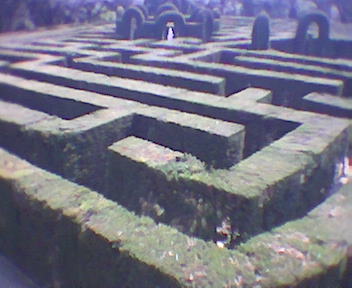This square photograph captures a slightly faded, somewhat dull, aerial view of an intricately designed garden maze. The maze, likely created from well-maintained hedges, features lush, green arches that form circular patterns throughout its layout. Although some parts of the maze appear covered in green moss, there are sections free of moss, suggesting varied maintenance. At the top of the image, in the center, there is a white object - possibly a person or statue - but its identity is unclear due to the photo's blur. In the background, a few rounded bushes add to the maze's natural elegance. There are no people visible in this photograph, and it lacks any identifying information or labels. The image appears to be taken during the day, though the lighting is subdued, and its relatively small size - around two by two inches - suggests it could be a snapshot intended for personal collection, potentially from a wealthy individual’s property or a museum display.